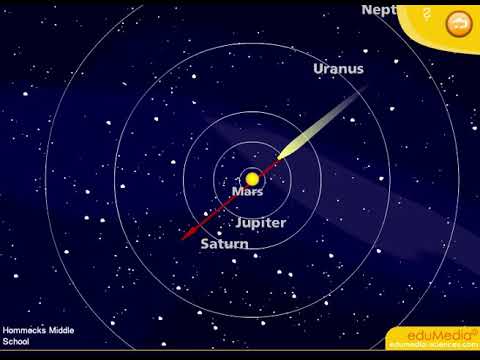This detailed image depicts a stylized map of outer space, focusing on the planets Mars, Jupiter, Saturn, Uranus, and Neptune. At the center, there's a yellow sphere labeled "Mars," encircled by several concentric rings. The innermost ring, marked "Mars," is followed by rings labeled "Jupiter," "Saturn," "Uranus," and "Neptune," radiating outward. A red rocket with a white plume extends through the central yellow Mars. The background is a deep navy blue, speckled with white dots resembling stars. In the lower left-hand corner, it is labeled "Hamex Middle School," while the lower right-hand corner features a yellow and white box saying "EDU Media," with an additional unreadable white text beneath it. Scattered colors of orange and brown can also be seen within the image.